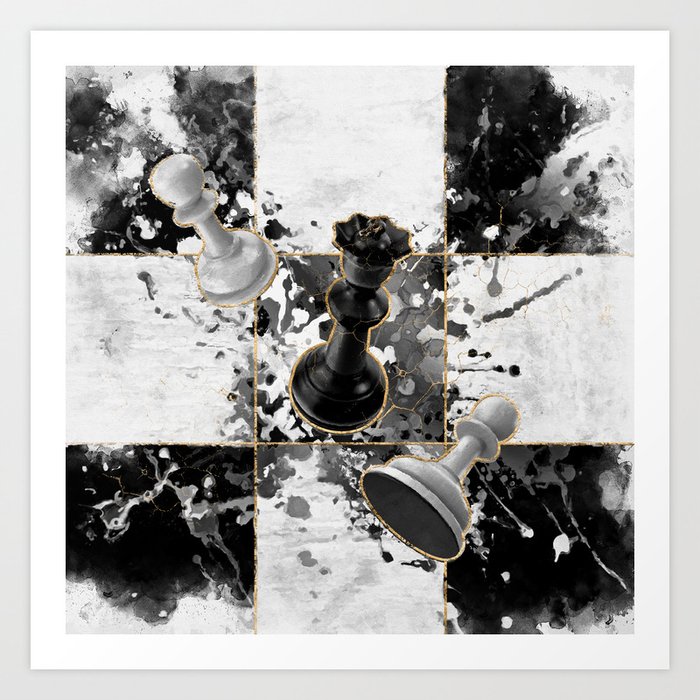This detailed black and white illustration showcases a partial chess board with nine squares, highlighted by an artistic, splattered-paint design. The board's marbled appearance features splotchy black and whitish gray marble for the squares, bordered by a distinct light gray outer and a thin white inner border. Each square is delicately outlined with a faint gold lining, adding elegance to the design. On the board, a commanding black queen occupies the center space, flanked by two white pawns—one lying on its side and the other angled towards the top left. The scene, appearing to be matted on a surface, juxtaposes the intricate marble-like texture with the lively chaos of splattered white paint.